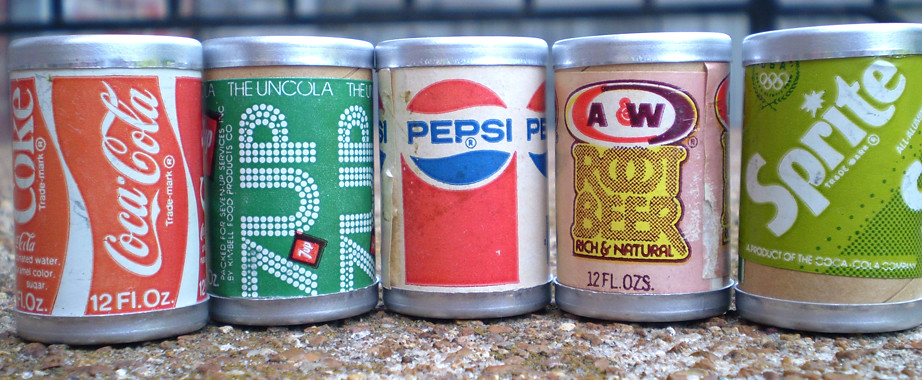In this image, we see five vintage soda cans lined up on a pebbled concrete surface, reminiscent of arm rails on public bridges. From left to right, the cans are Coca-Cola, 7 Up, Pepsi, A&W Root Beer, and Sprite. Each can features a distinct retro design and color scheme: 

1. The Coca-Cola can boasts a bright red background with white stripes and white lettering reading "Coca-Cola" and "12 fl oz" at the bottom.
2. The 7 Up can has a green background with white dots forming the words "7 Up, the Un-Cola."
3. The Pepsi can has a white background adorned with red shapes and blue lettering.
4. The A&W Root Beer can features a light pinkish background with yellow and brown text stating "Root Beer, Rich and Natural" and "12 fl oz," with the "A&W" logo in reds and browns.
5. The Sprite can is light green with white lettering that reads "Sprite," featuring a slightly brighter shade of green and vintage Olympic symbols.

Interestingly, these cans appear to be crafted from a combination of cardboard and metal, evidenced by a metallic top and bottom with cardboard-like bodies, enhancing their nostalgic appeal.